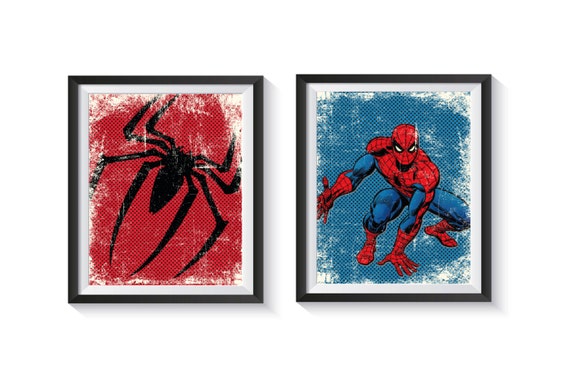This image showcases two framed pieces of Spider-Man-themed art hanging on a solid white wall. Both frames are rectangular and feature dark wooden frames, possibly walnut or ash, with white matting around the edges. The artwork inside the frames aligns with a distressed, vintage comic book aesthetic.

The piece on the left highlights a red, distressed background with white scratches and a prominent, stylized black spider emblem with elongated, pointy legs in the center, suggestive of a close-up from Spider-Man's uniform. The right piece features a similarly distressed blue background. This artwork portrays Spider-Man in his iconic red and blue suit, crouched down with one hand on the ground and the other extended forward, as if reaching out of the frame. His muscular form and determined gaze are captured with the classic black webbing pattern and large white eyes on his mask, emphasizing his dynamic and legendary pose. The texture and wear on both pieces contribute to their nostalgic, comic-book feel.